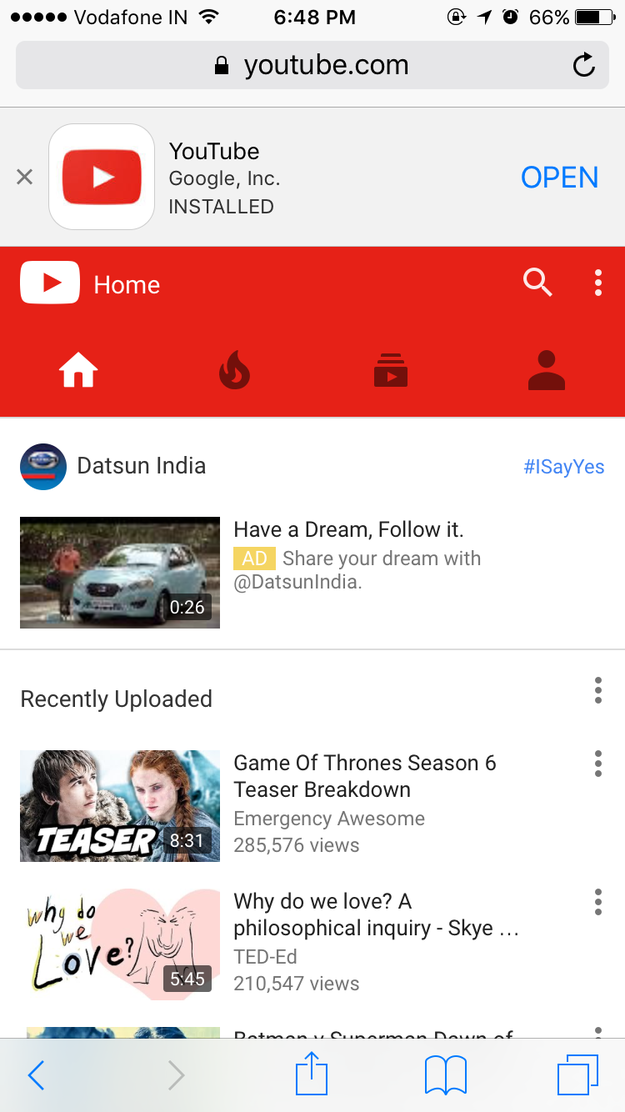Here is a cleaned-up and detailed caption for the described cell phone screenshot:

The screenshot captures a cell phone display with several distinct elements. 

- **Top Bar**:
    - The very top section is black, featuring the current time, battery percentage, and signal reception icons aligned from left to right.

- **Browser Toolbar**:
    - Below this is a centered gray rectangle, likely the address bar, with a black padlock icon to its right and the text "youtube.com." 
    - A reload arrow icon is situated on the far right of this toolbar.

- **YouTube Interface**:
    - Beneath the browser toolbar is another rectangle; the top half is gray, and the bottom half is red.
    - On the gray left section, there's a white square containing a small red rectangle with a white arrow pointing to the right.
    - To the right of this icon, the text reads "YouTube Google, Inc installed."
    - On the far right edge, the word "OPEN" is displayed in all caps in blue.

- **Red Navigation Bar**:
    - In the red section, there's a white rectangle in the upper left corner containing another red right-pointing arrow.
    - The word "Home" is displayed in white next to it.
    - Towards the right, there’s a white magnifying glass icon, followed by a vertical ellipsis (three dots).

- **Advertisements and Content**:
    - Below the red navigation bar, the bottom half of the screen features various icons and advertisements.
    - The central ad highlights "Dots in India," showing an image of a white car on the left. To its right, the text reads, "Have a dream, follow it."
    - Below this ad, the section "Recently Uploaded" lists videos:
        - The first video is a "Game of Thrones Season 6 Teaser Breakdown," represented by a clickable rectangular thumbnail on the left.
        - Below it, another clickable rectangle leads to the video "Why Do We Love? A Philosophical Inquiry."

This cleaned-up caption provides a detailed and organized description of the cell phone screenshot, capturing all key elements and their positions.